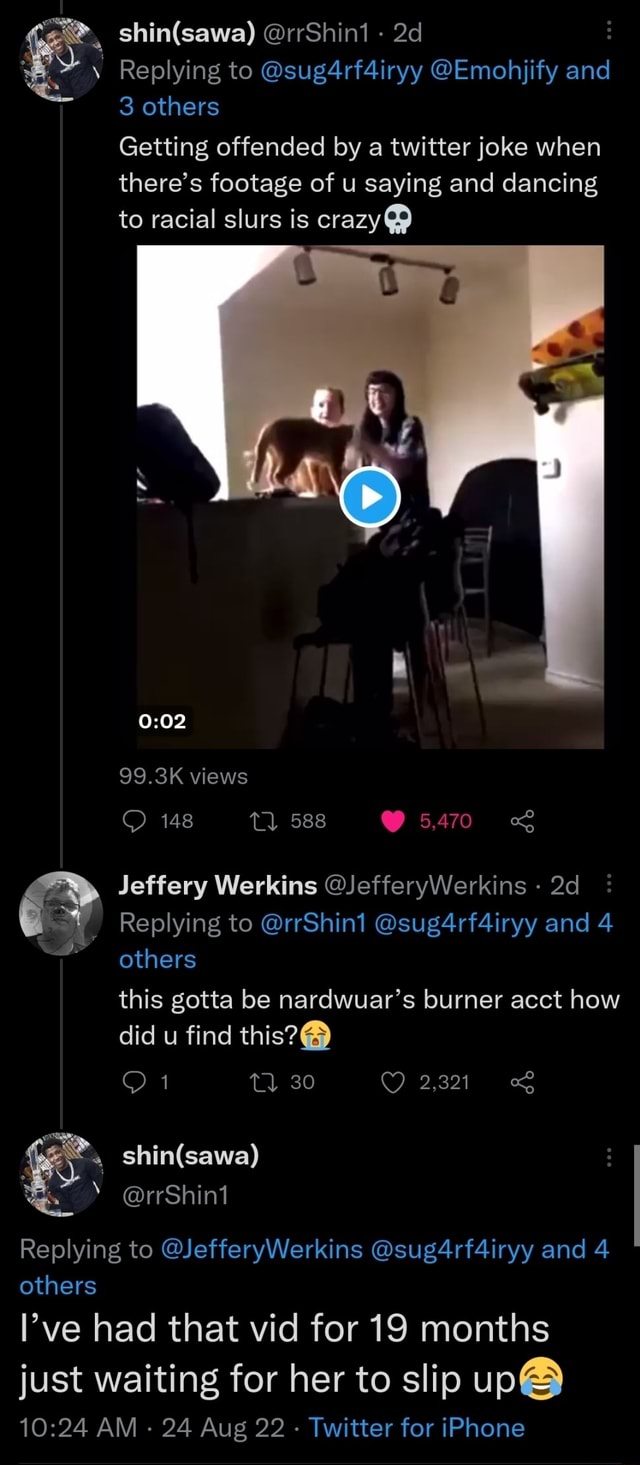This image is a screenshot of a Twitter conversation displayed on a black background. At the top, there is a profile picture featuring rapper NBA Youngboy, belonging to a user named Shin Sawa whose handle is @rrshin1. Shin Sawa replied to a conversation involving a user named Sugar Fairy and others. The tweet reads: "Getting offended by a Twitter joke when there's footage of you saying and dancing to racial slurs, it's crazy." Attached to this tweet is a two-second video that has garnered 99.3 thousand views, 140 comments, 588 retweets, and 5,470 likes.

In the replies, a user named Jeffrey Workings comments, "This gotta be Nardwuar's burner account, how did you find this?" accompanied by a crying laughing emoji. Shin Sawa responds, "I've had that vid for 19 months just waiting for her to slip up," also adding a crying laughing emoji to their reply.